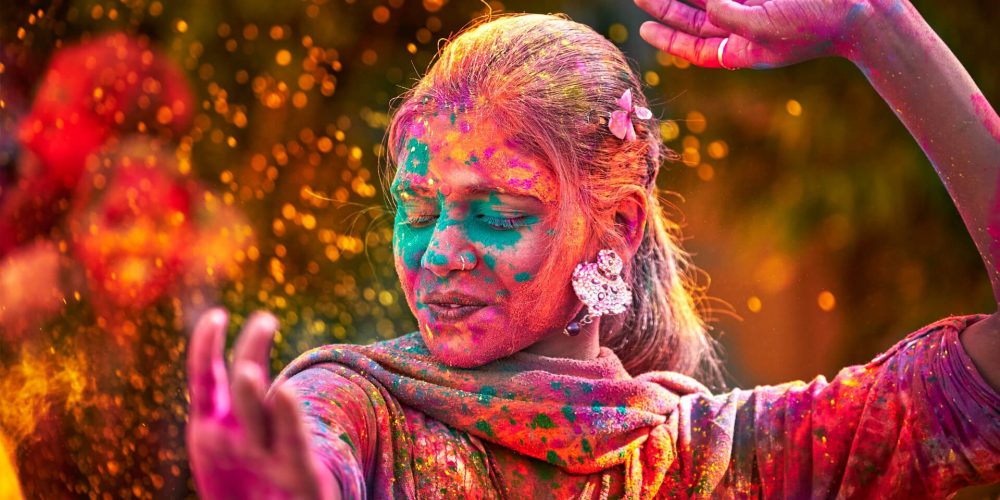A vibrant and dynamic image captures a young woman seemingly dancing in the midst of a lively festival. Her skin is painted a striking purple, adorned with sparkles, and her face is splattered with various colors of paint—blues, yellows, pinks, and greens. She's dressed in a multicolored outfit and wears a scarf around her neck, along with large silver earrings and a ring on one raised hand. Her blondish hair is pulled back, and she appears to be moving with one hand extended in front of her and the other raised. The background is filled with blurred faces also covered in paint and what looks like colorful lights or paint being thrown, adding to the festive atmosphere. The image is a professional photograph that bursts with color and energy, capturing the essence of celebration and joyful chaos.